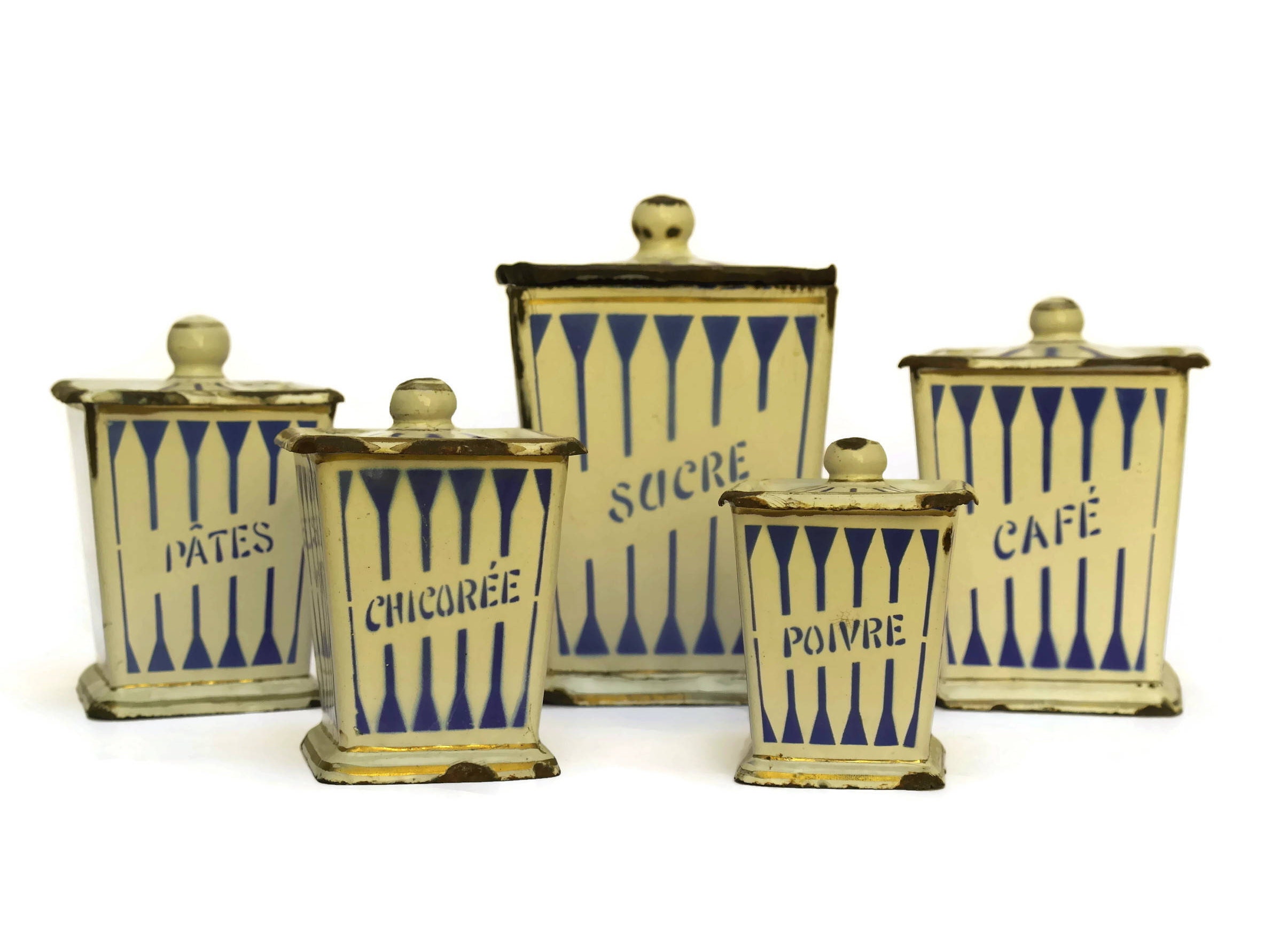This image features a collection of five antique-looking, rectangular canisters with trapezoidal hints, set against a white background. The canisters, appearing somewhat aged with wear on the corners and bottom, are primarily a light yellow color with blue stripes. Each canister has a matching lid topped with a small, doorknob-like handle, enabling easy removal. The containers are labeled in French with blue text, facing forward. From left to right, the labels read "pâtés," "chicorée," "sucre" (which means sugar), "poivre," and "café," possibly indicating their intended use for coffee preparation.